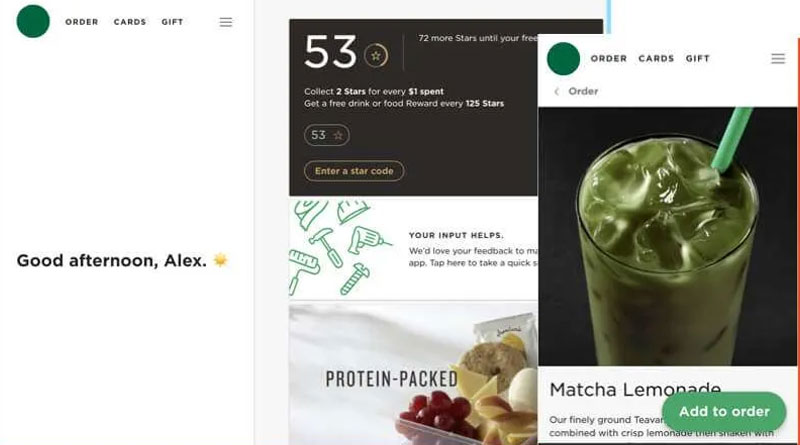The image depicts a webpage featured prominently. On the left third of the picture, the top left corner displays a green circle. Adjacent to this are three clickable menu items labeled "Order", "Cards", and "Gift". To the far right of these menu items, there is a three-dot menu icon, all set against a white background. Centrally aligned in this portion is the greeting "Good Afternoon, Alex" in black text, accompanied by a yellow sun emoji, also on a white background.

Moving to the right third of the picture, the same website shows details of a "Matcha Lemonade" listing. At the bottom right is a green "Add to Order" button with white font. The description for the Matcha Lemonade starts with "Our Friendly Ground, a Teavana..." but the rest is obscured by the "Add to Order" button. Partial visible text continues with "...combined with Chris Lemonade, then shaken with...," though it is cut off at the bottom of the webpage.

Above the description is an image of the Matcha Lemonade in a clear cup with a green straw, showcasing a green drink. The top portion features both an "Order" button and a "Back" button above the picture.

Centered within the image is a feedback block titled "Your Input Helps, We'd Love Your Feedback." Below this section appears an image of a fruit and cheese plate labeled "Protein Pact".